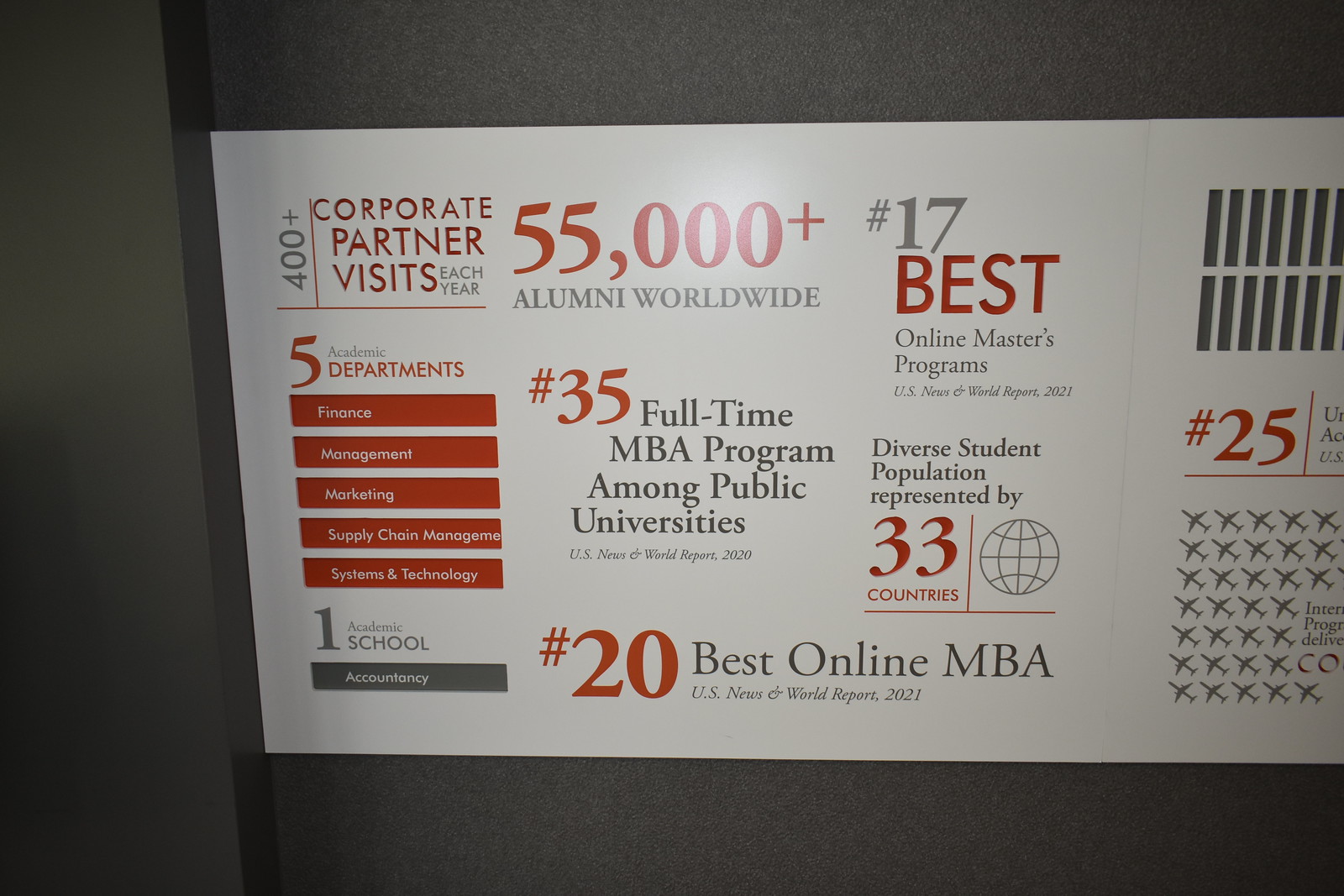The image depicts a landscape-oriented color photograph of a rectangular poster adhered to a dark gray wall or door. The poster, with white, red, and gray text, highlights the achievements and rankings of an educational institution. The left section prominently displays text stating, "400+ corporate partner visits each year" in dark red, while directly adjacent larger red text declares, "55,000+ alumni worldwide." Below this, it lists "five academic departments" in white text on a red background, as well as mentioning "one academic school" and "35 full-time MBA program among public universities."

Additionally, the poster features rankings distributed throughout its layout, such as "20 Best Online MBA" and "17 Best Online Master's Programs," with these accolades attributed to "U.S. News and World Report 2021" and "2011," respectively. Positioned in columns, with varied text sizes and graphical elements like cut-off images of small airplanes, the text composition emphasizes the accomplishments in a clear and structured manner. This detailed visual representation underscores the institution's national and international stature in academia and professional partnerships.